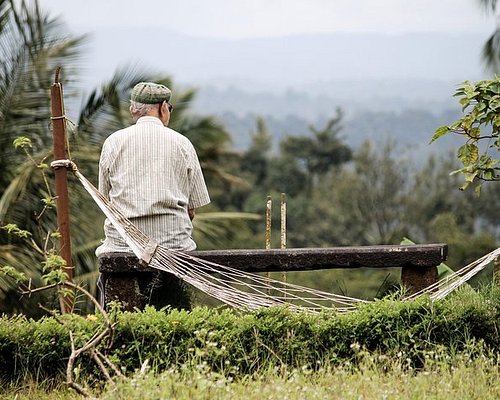In this daytime photograph taken from a scenic park, an older gentleman is seen sitting on an aged stone bench with his back to the camera. He is dressed in a white short-sleeved, button-down shirt, donning glasses and a green hat atop his gray hair. The bench is positioned to the left middle ground of the image, in front of a hammock suspended from bamboo posts. The lush surroundings are vibrant with greenery, including grass, trees, and various plants. Bushes scatter the scene, adding density to the green environment. The setting appears humid and cloud-covered, with sunlight diffused through the overcast sky. In the distance, the landscape transitions to a hazy valley filled with tropical vegetation, with layers of hills and mountains forming a faintly silhouetted horizon. The gentleman appears to be quietly soaking in the tranquil and expansive view.